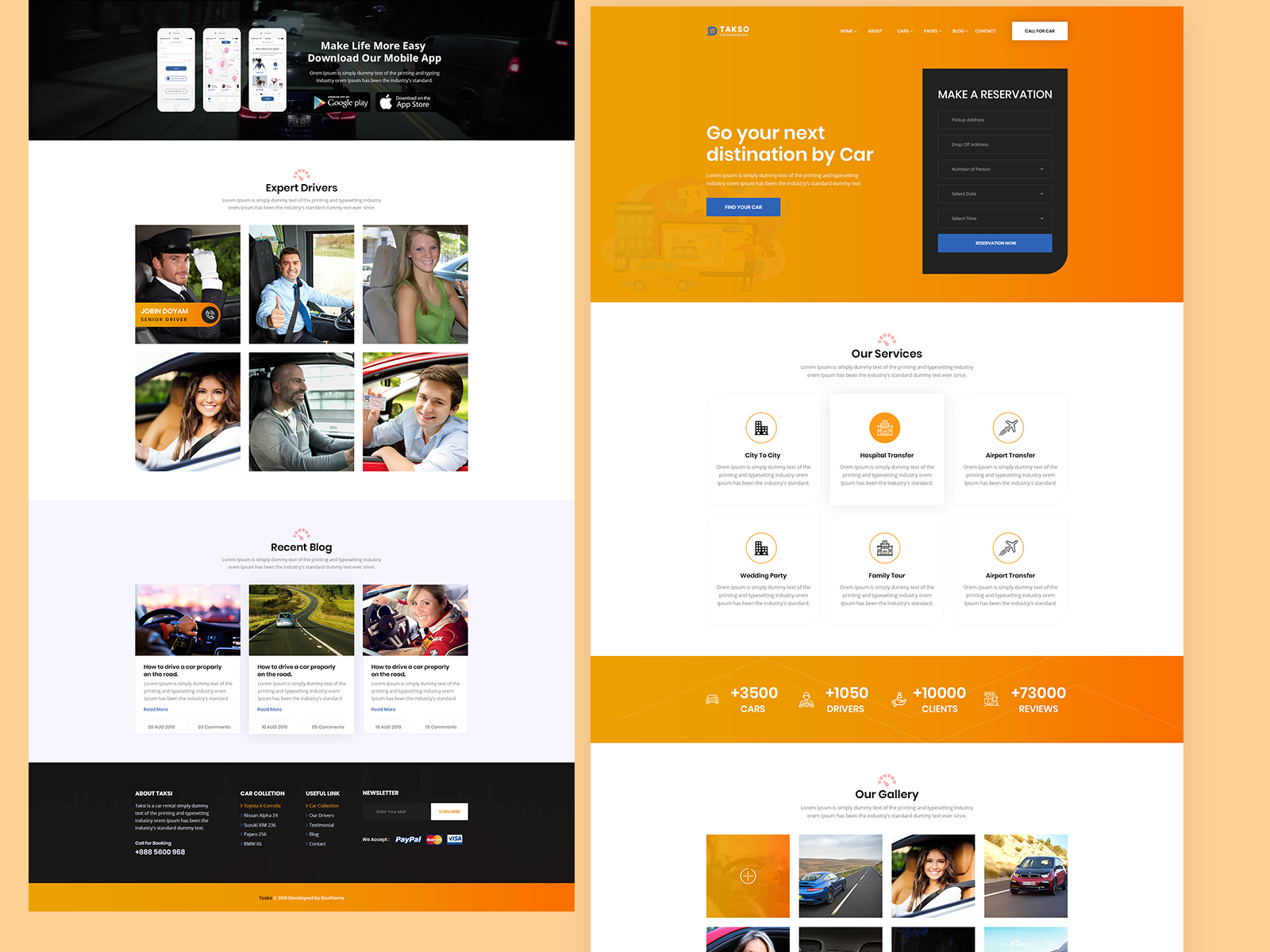The image displays two smartphone screenshots placed side by side. 

The screenshot on the left features a white main area framed by black bands at the top and bottom. Central text reads "Expert Drivers," followed by two rows of three square photographs each, depicting individuals seated behind the wheels of cars. Below this section, a heading titled "Recent Blog" is displayed with three landscape images: one showing a person steering a car from behind, another portraying a car on an open countryside road, and the third capturing a woman who appears to be a race car driver sitting at the wheel.

The screenshot on the right showcases an orange background with white stripes. The top orange band contains the text, "Go your next destination by car," below which is a black square with the text "Make a Reservation." The subsequent white stripe lists "Our Services," organized into two rows of three icons each, representing "City to City," "Hospital Transfer," "Airport Transfer," "Wedding Party," "Family Tour," and "Airport Transfer." The bottom section features an orange bar with service statistics: "3500+ cars," "1050+ drivers," "10,000+ clients," and "73,000+ reviews."